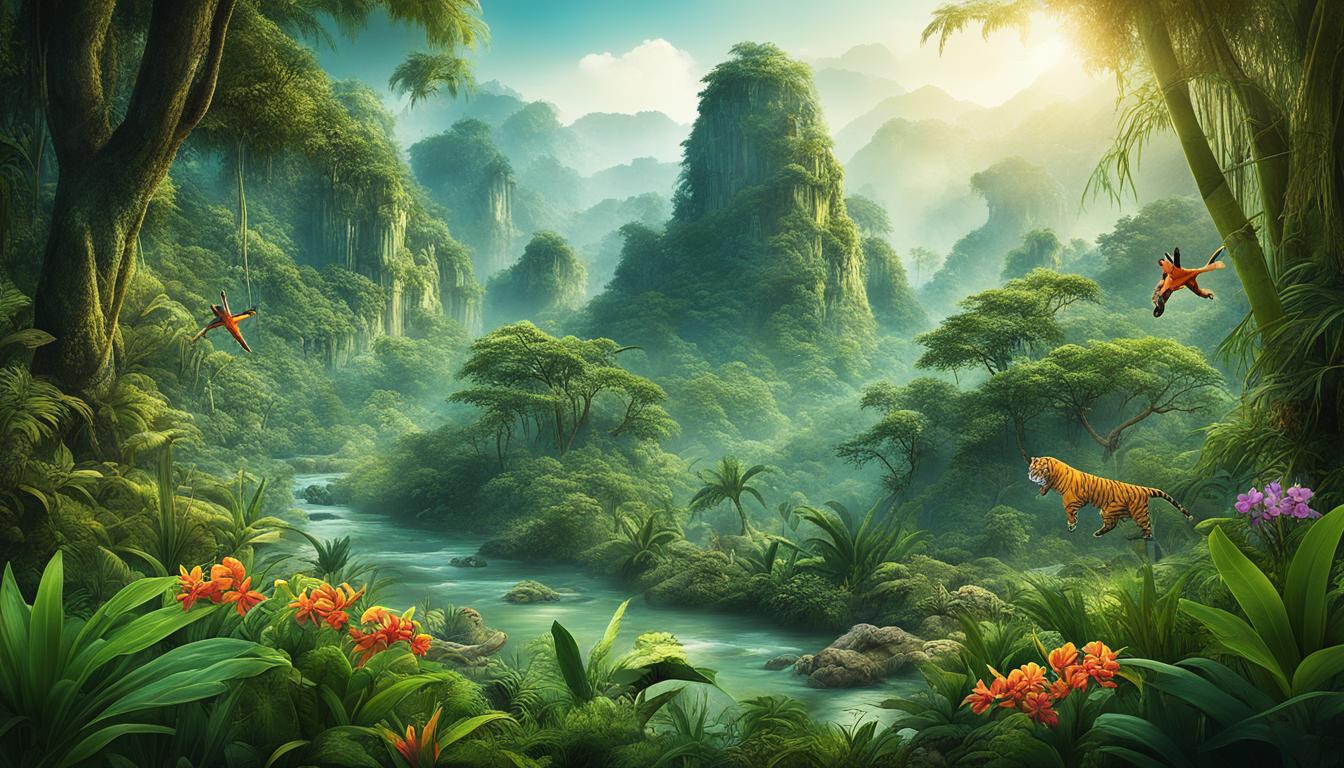The painting depicts a lush and magical jungle scene with a soft, almost dreamlike quality. Dominating the center of the composition is a teal-colored stream with rocks and lilies lining its edges. To the left of the stream stands a large tree with a gnarly trunk, around which a vibrant orange bird is fluttering. The scene is bathed in soft light, with fluffy, rolling clouds receding into a light blue sky, and the sun shining brightly from the right-hand side.

On the right side of the stream, a diversity of trees and foliage flourishes, including various leaves of different sizes. Nearby, an elegant tiger with striking orange and black stripes appears to be leaping towards the water, its darker tail trailing behind. Coral and purple flowers, along with other orange blossoms, add splashes of color near the water's edge. Above the tiger, another orange bird can be seen soaring through the dense growth, enhancing the sense of vibrant biodiversity.

In the distance, the forest continues to thrive, with green bushes and oval-shaped plants contributing to the lush, verdant atmosphere. The overall scene captures the wild beauty and dynamic vitality of a healthy rain forest ecosystem.